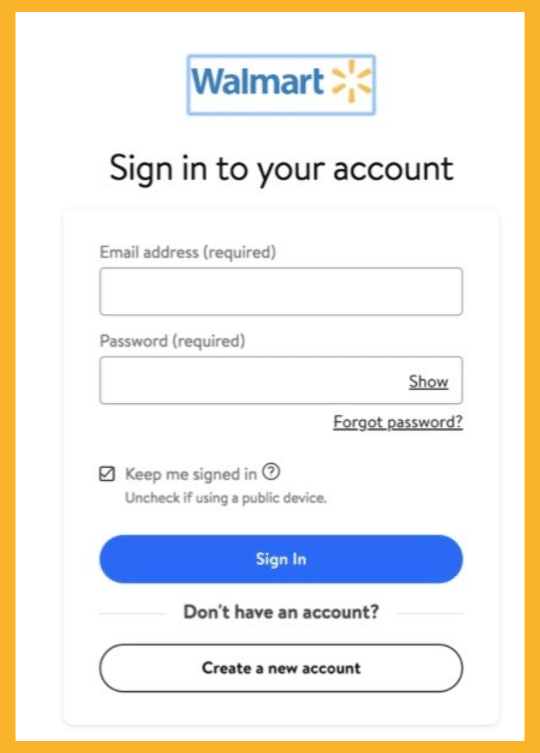The screenshot captures a Walmart sign-in window, primarily used for logging into the Walmart.com website. Dominated by a clean and user-friendly interface, the center of the image prominently features the word "Walmart" written in blue and enclosed within a blue-outlined box. At the very top and center of the window, the familiar Walmart logo is displayed alongside the company's name.

Beneath the brand name, large black text reads "Sign in to your account," guiding users to the login fields below. The login section includes two input fields: one for the email address and another for the password. Positioned below the password field is a "Forgot password?" link, offering an option for users who need to recover their account details. 

A checkbox labeled "Keep me signed in" is prominently checked, ensuring users remain logged in during subsequent visits. At the bottom of this section is a striking blue "Sign-In" button meant to facilitate the login process.

Further down, the window addresses users who do not yet have an account. The text "Don't have an account?" is followed by a "Create a new account" button, providing a seamless link for new user registrations.

Overall, the sign-in section is distinctly boxed with an orange outline, visually segregating it from the rest of the website content. This screenshot only illustrates a portion of Walmart's website, concentrating on the streamlined and functional design of the sign-in process.